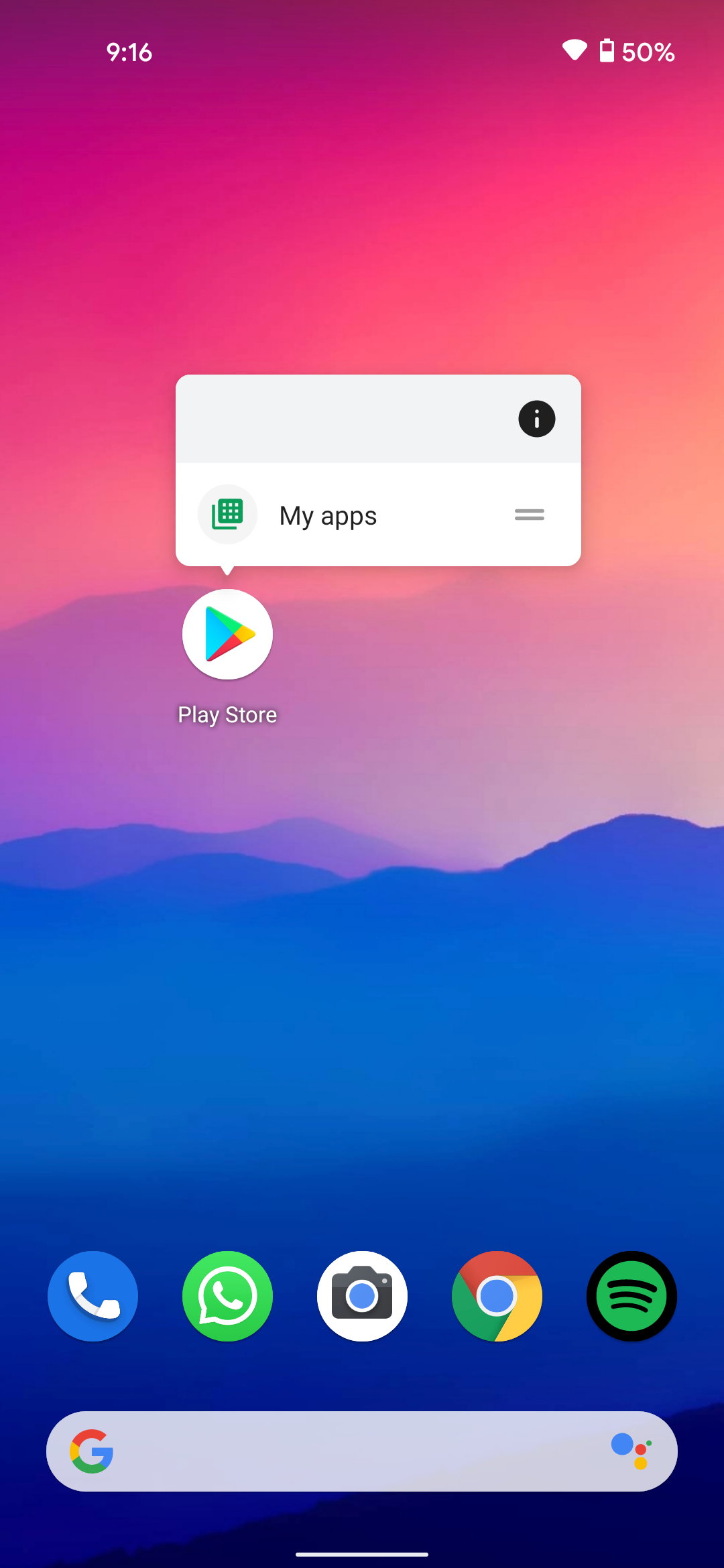The image is a detailed screenshot of a smartphone’s home screen with an abstract background that visually transitions from darker shades to lighter ones. At the bottom, the background depicts a mountain range in various shades of blue, which gradiently shifts to light lavender mid-screen. Further upwards, the lavender mixes into soft hues of pink and orange, climaxing in a deep purple at the very top.

In the upper left corner, the time is displayed as "9:16." The upper right corner shows the battery icon, indicating a 50% charge, alongside the Wi-Fi signal icon. Centrally located is a prominent white rectangle bordered by a thin light gray line. At the top-right corner of this rectangle, there is a black circle containing a white inverted "i", symbolizing information. Just below this border, the text "My Apps" is displayed.

Within the rectangle, the Play Store logo is visible; it consists of a white circle encompassing a multi-colored pyramid shape. Below this logo, in small white font, is the text "Play Store."

At the bottom of the screen, there are five icons: a blue phone icon, a green WhatsApp icon, a camera icon, a Google Chrome icon, and a green Spotify icon. Below these, the Google search box is prominently displayed as a white rectangle with rounded corners. The iconic "G" logo of Google appears on the left side, while on the right, there is a smaller search logo featuring a blue circle beside a tiny red circle, complemented by a slightly larger yellow circle.